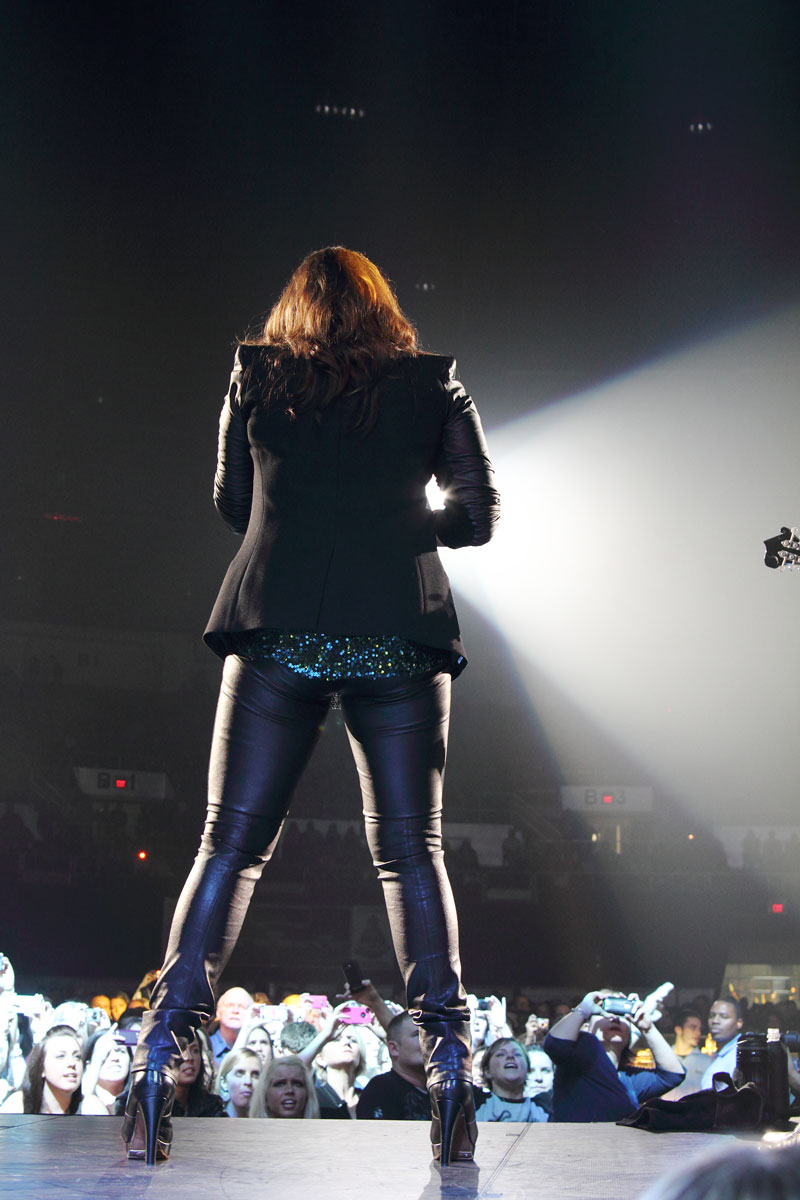In the photograph, a woman is seen from behind as she performs on a stage, which occupies the bottom portion of the image. The stage itself is a solid black, raised platform. She stands confidently, dressed in black leather, ankle-high high-heeled boots, and tight black leather pants. Over this, she wears a black fabric jacket, beneath which a blue sequin shirt shimmers. Her brownish-red hair flows naturally, adding to her striking presence.

The audience's heads are visible, close to the stage, all attentively looking up at her. Beyond them, tiered seating fades into the background, filled with more spectators. The ceiling is illuminated by multiple lights directed towards the stage, spotlighting her and enhancing the overall ambiance. The room is predominantly dark except for these focused lights and some subtle red lights farther off. Though her hands are partially visible up to the elbow, they seem to be holding a microphone, completing the scene of a captivating live performance.